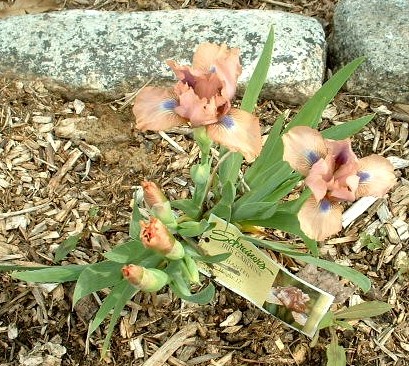This image features a photo of peach-colored roses, possibly bordered by other flowers of a similar hue. The flowers are planted amid a mix of brown dirt, burnt grass, and wood chips. Surrounding the flowers are gray and white stones that serve as a border for the flower bed. The flowers stand upright with green leaves, each rose opening up into three petals with a distinct central purple dot. A visible tag is present among the flowers, although the text is too small to read, presumably identifying the flower species. The photo appears to have been taken outdoors in a garden or along a walkway during the daytime, from a vantage point looking down on the flowers, suggesting the photographer was either standing or kneeling.